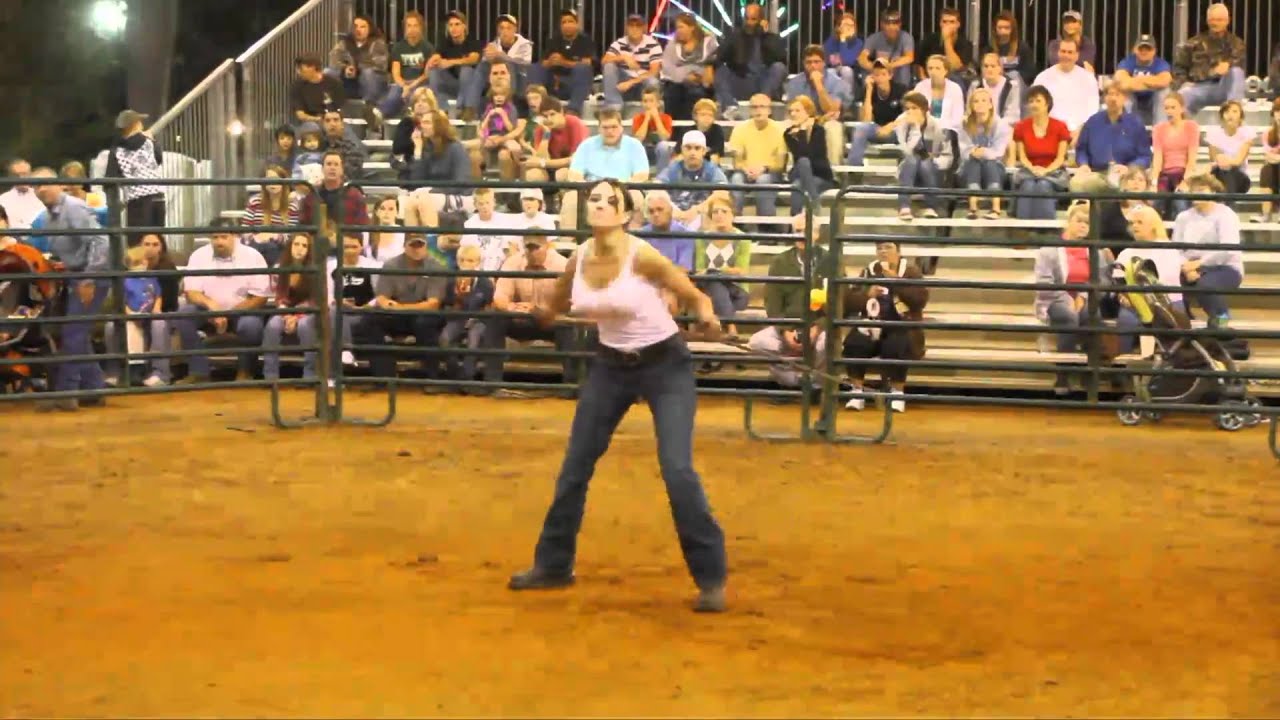In a slightly blurry photograph set in an indoor bull riding arena, a woman stands at the center of a dirt-covered ring, surrounded by metal fences. The ground is a distinct yellowish, copper-ray hue, typical of rodeo settings. The metal bleachers, which arc around the perimeter of the arena, are populated by spectators, many dressed in jeans. At the horizon of this dimly lit scene, a Ferris wheel can be vaguely seen against the nighttime sky, adding a whimsical touch.

The woman, dressed in dark jeans, boots, and a white crop top, has brown hair tied in a ponytail, some strands obscuring her face. She faces the camera but isn't looking directly at it, suggesting a moment perhaps caught off-guard or in the middle of activity. To either side of her are baby strollers, hinting at a family-friendly atmosphere. Most onlookers appear engaged, suggesting she might be performing, possibly dancing or involved in some aspect of a local bull-riding show. The soft arena lights cast gentle shadows, reinforcing the sense of a small, local gathering.